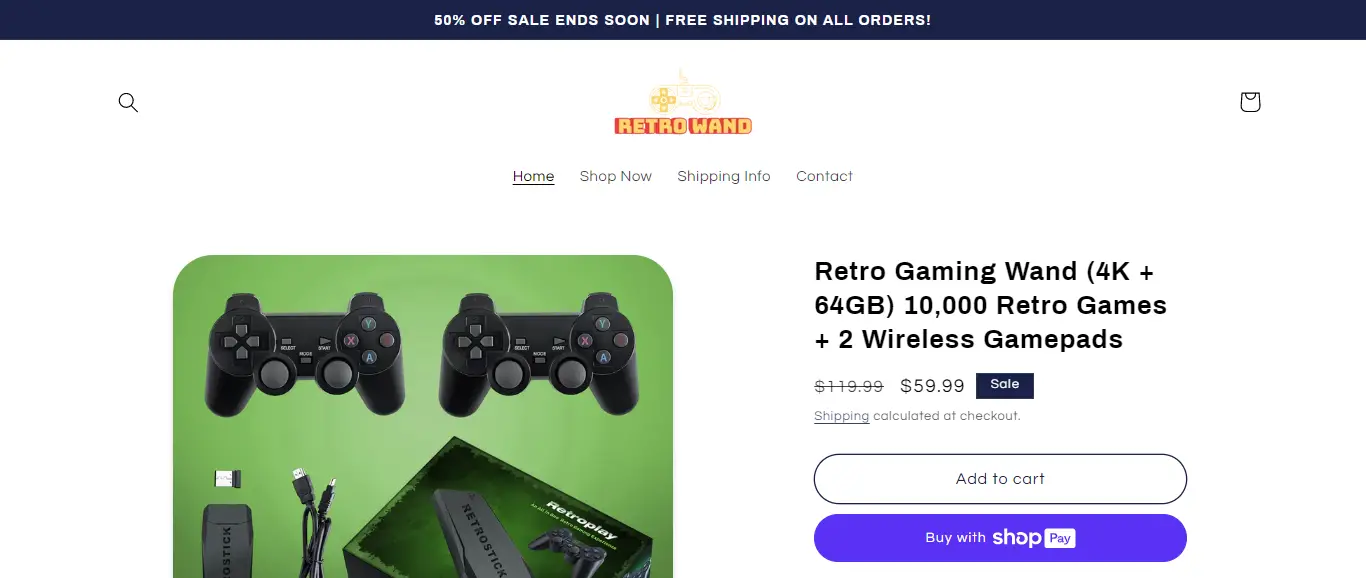The image depicts a section of a retro-themed shopping website. At the very top center, bold white text announces a "50% off sale" and "free shipping on all orders." Below this announcement, the site’s logo, "Retro Wand," is displayed in an orange, retro-styled font with darker orange shading. Adjacent to the logo, there is a light yellow controller icon. On the far left, a magnifying glass icon is visible, signifying the search function. Opposite on the far right, a mail icon is displayed.

Directly underneath the logo, four navigation categories are listed: "Home," "Shop Now," "Shipping Info," and "Contact." 

At the bottom left, there is a photograph featuring two black PlayStation 3 controllers against a green background. The image also shows additional accessories, including a cord and a Bluetooth dongle. To the right of this photograph, the product name "Retro Gaming Wand" is prominently displayed alongside a 50% discounted price of $59.99.